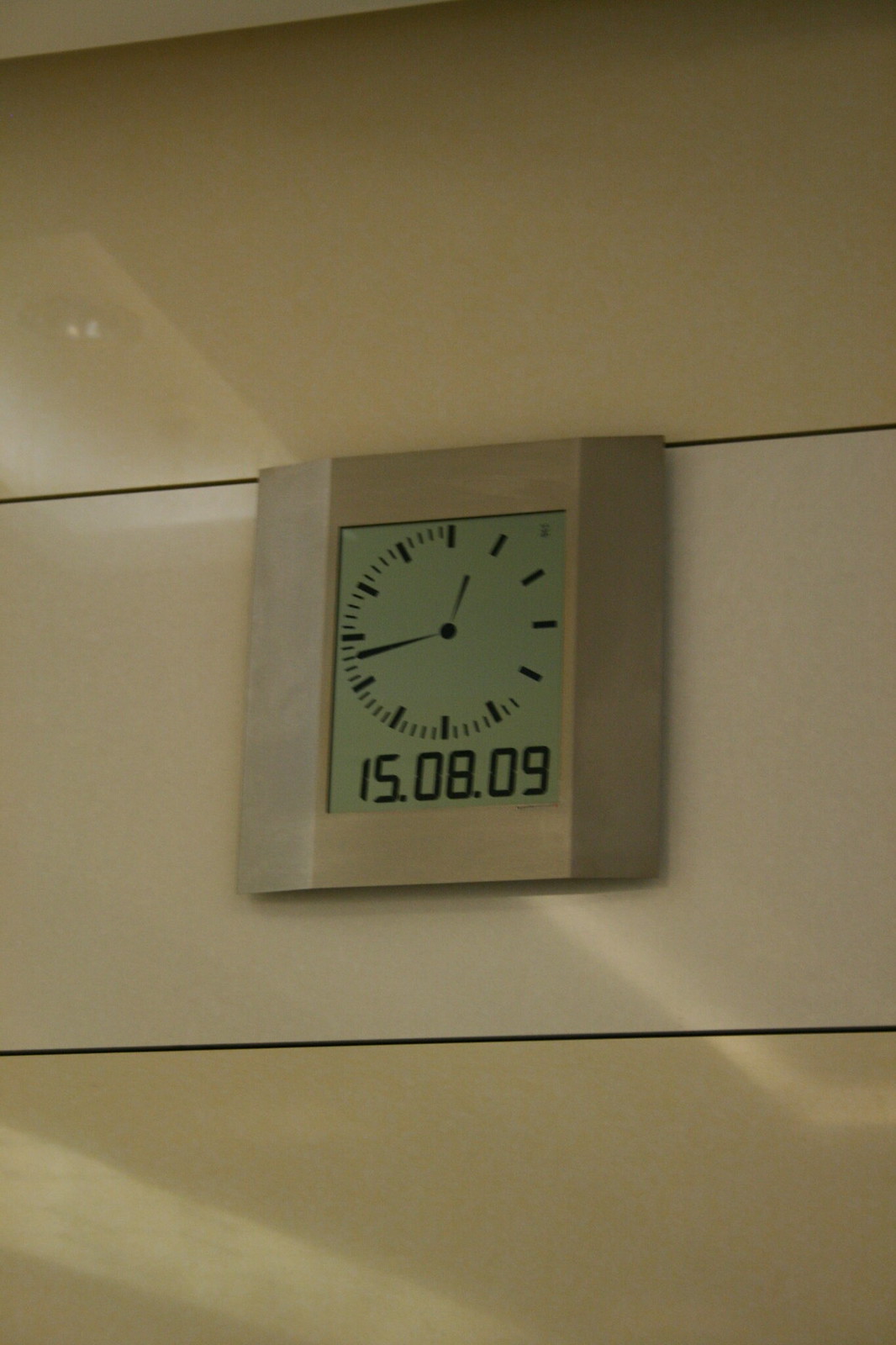This is a detailed photograph of an early, simple digital clock with a thick silvery frame, hanging on a wall. The clock face is minimalist, featuring only dashes instead of numbers to mark the hours. The hands of the clock, both resembling baseball bats without handles, show the time as slightly before 1 o'clock and 43 minutes past the hour, suggesting it is 12:43. Underneath the analogue display, the screen shows black numerals reading "15.08.09," which could be interpreted as a date. The clock is mounted on a wall with a light yellow and white background that is divided horizontally into three sections by two black lines, giving the wall a structured appearance.